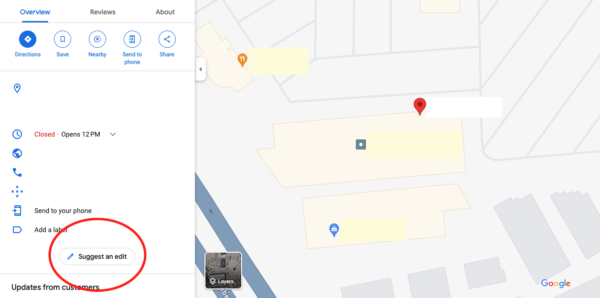The image is a screenshot of a Google search result page. At the top left corner, three distinct categories can be seen: "Overview," "Reviews," and "About." Just below these categories, a series of action buttons are displayed, labeled as "Directions," "Save," "Nearby," "Send to Phone," and "Share." The name of the place in question has been intentionally crossed out, concealing its identity. However, it is visible that the place is currently closed and is scheduled to reopen at 12 PM. At the bottom of the screen, a red oval highlights a button labeled "Suggest an Edit," drawing attention to this option for users.